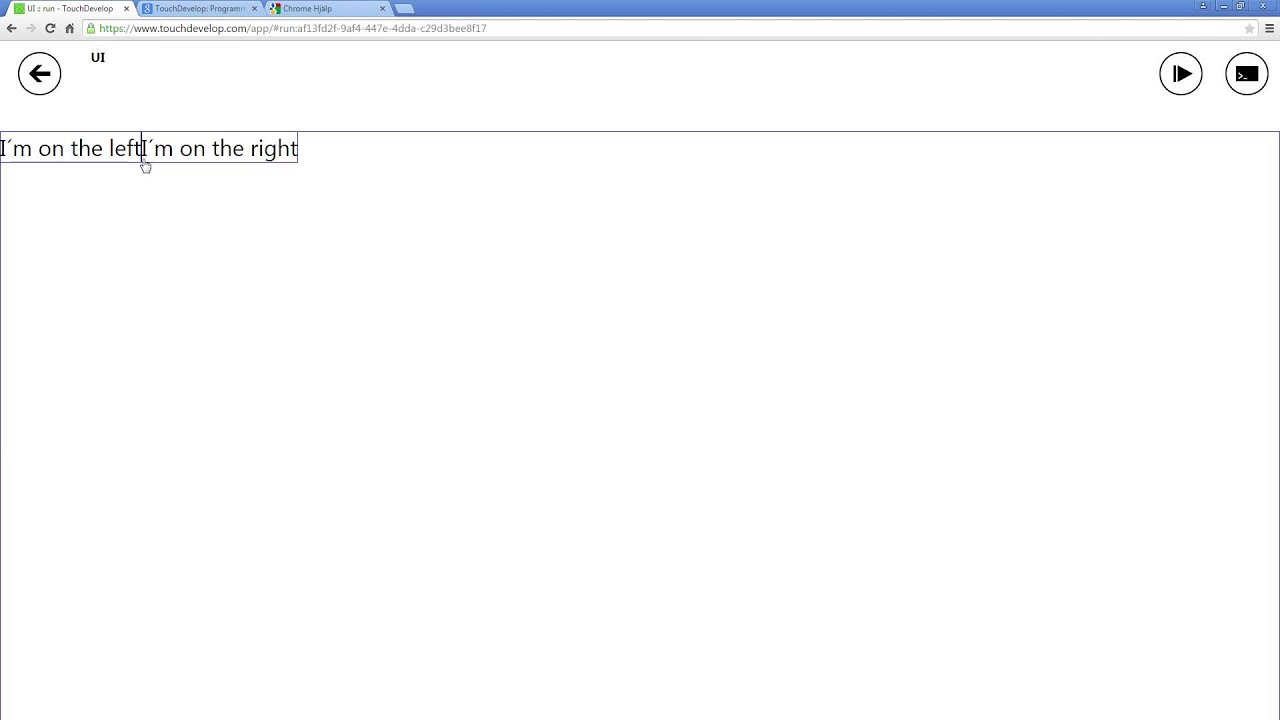A detailed screenshot of a computer monitor displaying three browser tabs is open. The active tab is titled "Tour Develop" or "Travel Develop." The other two tabs are "Google Chrome Help" and "Check Desktop Progress." Just below the tabs, the browser's navigation bar features a left-facing arrow, a refresh button, a Home button, and an address bar. To the far right of the address bar is a hamburger menu icon. 

Beneath the navigation bar is a white section containing a circled left-facing arrow followed by the uppercase letters "UI." Toward the far right of this white section, there are circular Play and Stop buttons. Further down, the screen shows a text area with a cursor positioned between the words "left" and "I'm" from the phrases "I'm on the left" and "I'm on the right." The absence of a space between "left" and "I'm" suggests that the user is in the process of editing this text to input a space or punctuation.